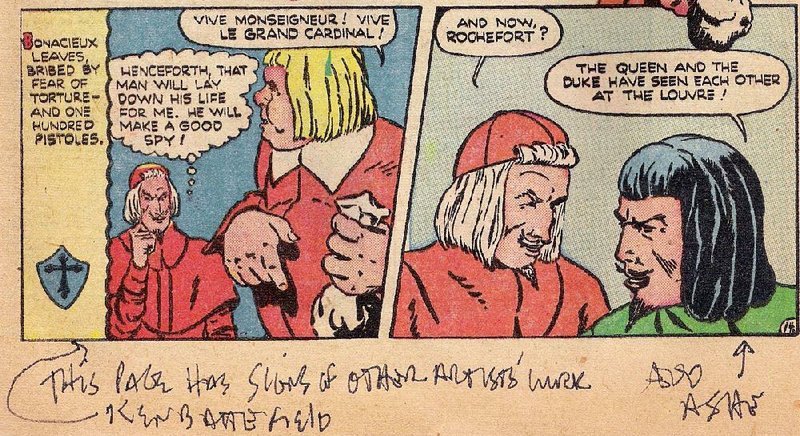This image is a comic strip composed of two distinct cartoon frames, each featuring characters in historical attire, suggesting a setting from medieval or Renaissance times. The first frame portrays two men in conversation. Dominating the scene is a man dressed in a cardinal's red robes, complete with a red shawl, a round red cap, and long white hair. In a thought bubble above his head, he muses, "Henceforth, that man will lay down his life for me. He will make a good spy." Opposite him stands a man with straight-cut blonde hair, holding a white bag, who exclaims, "Viva Monsieur, Viva Le Grand Cardinal." Text alongside this panel reads, "Bonacieux leaves bribed by fear of torture and 100 pistoles."

The second frame continues with the cardinal, now addressing a new character named Roquefort. This new figure, with long black hair, a goatee, and dressed in a green shirt, informs the cardinal, "The Queen and the Duke have seen each other at the Louvre." Background elements, including a light brown tan backdrop and a shield with a cross, contribute to the period-appropriate atmosphere. Handwritten at the bottom of the page, albeit difficult to decipher, is a note suggesting, "this page has signs of other artists' work."

Together, these elements create a narrative rich in intrigue and historical detail, highlighting covert schemes and loyalty within a grand, courtly context.